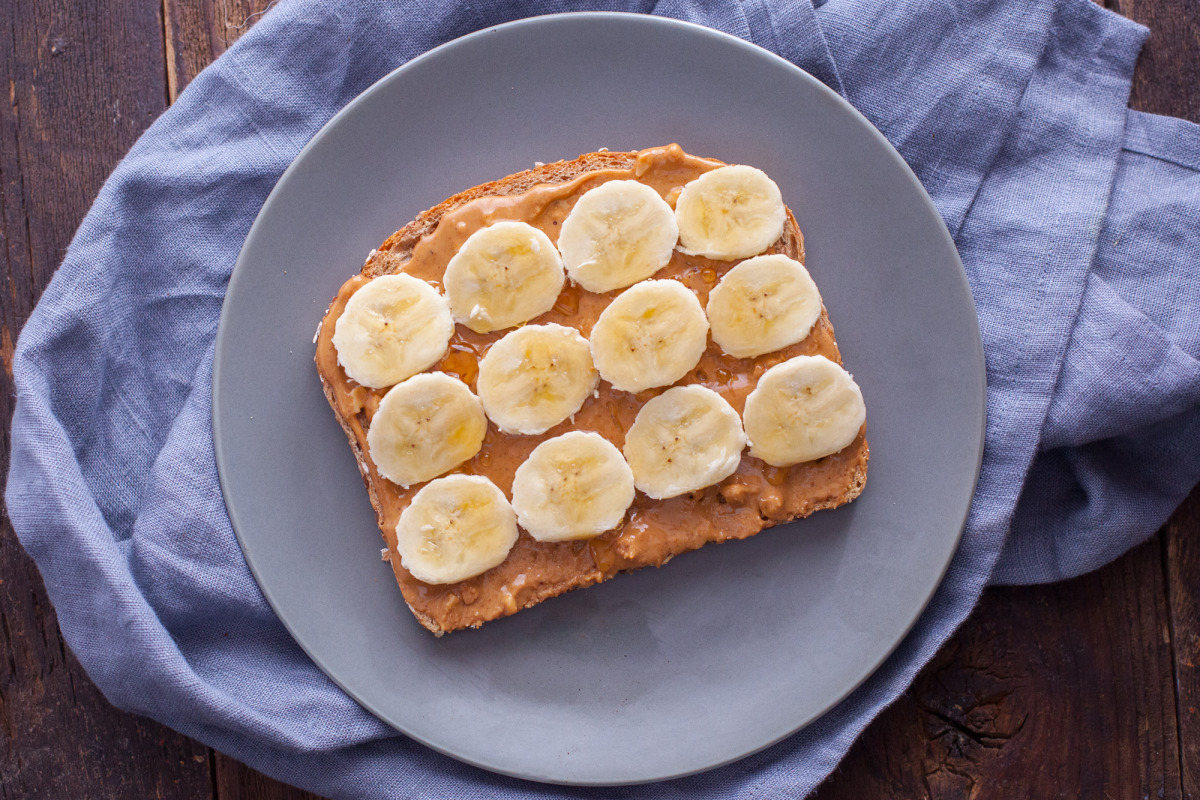This image captures a visually appealing and appetizing open-face peanut butter and banana sandwich situated on a blue ceramic plate. The plate rests on a slightly crumpled, blue cotton towel atop a solid wooden table. The sandwich features a slice of whole wheat bread generously spread with chunky peanut butter, evident by the visible pieces of peanuts within the spread. Carefully arranged on the peanut butter are 12 banana slices, neatly organized into three rows of four slices each. To add a touch of sweetness, the sandwich is drizzled with honey. The vibrant composition, with its consistent blue hues and warm wooden backdrop, makes the setting pleasing and inviting.